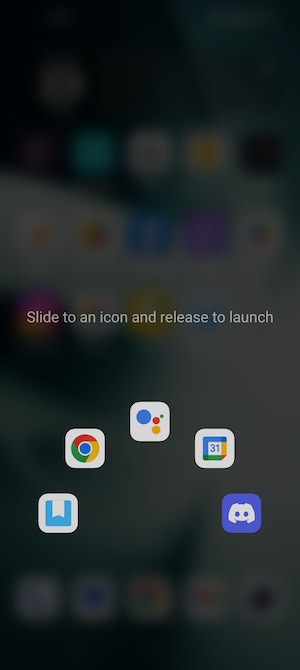The image depicts the launch page on a smartphone, characterized by a predominantly dark, almost black background. Faint outlines of various app icons are visible, obscured by the dark overlay. Central to the image, the text reads, "Slide to an icon and release to launch." Below this, five app icons are arranged in a slight arc, beginning at the bottom left and extending upwards before curving back down to the bottom right.

Starting from the left, the first icon is a white square displaying a prominent blue "W," though its exact application is unclear. The next icon, moving upwards, is a white box containing the recognizable Google Chrome logo, featuring a blue circle at the center encircled by red, green, and yellow segments. At the apex of the arc, the third icon displays the Google Assistant logo, characterized by a large blue dot, smaller green dots, and even smaller red and yellow dots.

To the right, the fourth icon is the Google Calendar symbol, shown as a white square with a multi-colored, bent-corner design—blue, green, yellow, and red—with the number "31" at the center. Finally, at the bottom right, there is a blue square displaying a stylized game controller, though its specific application remains unidentified.